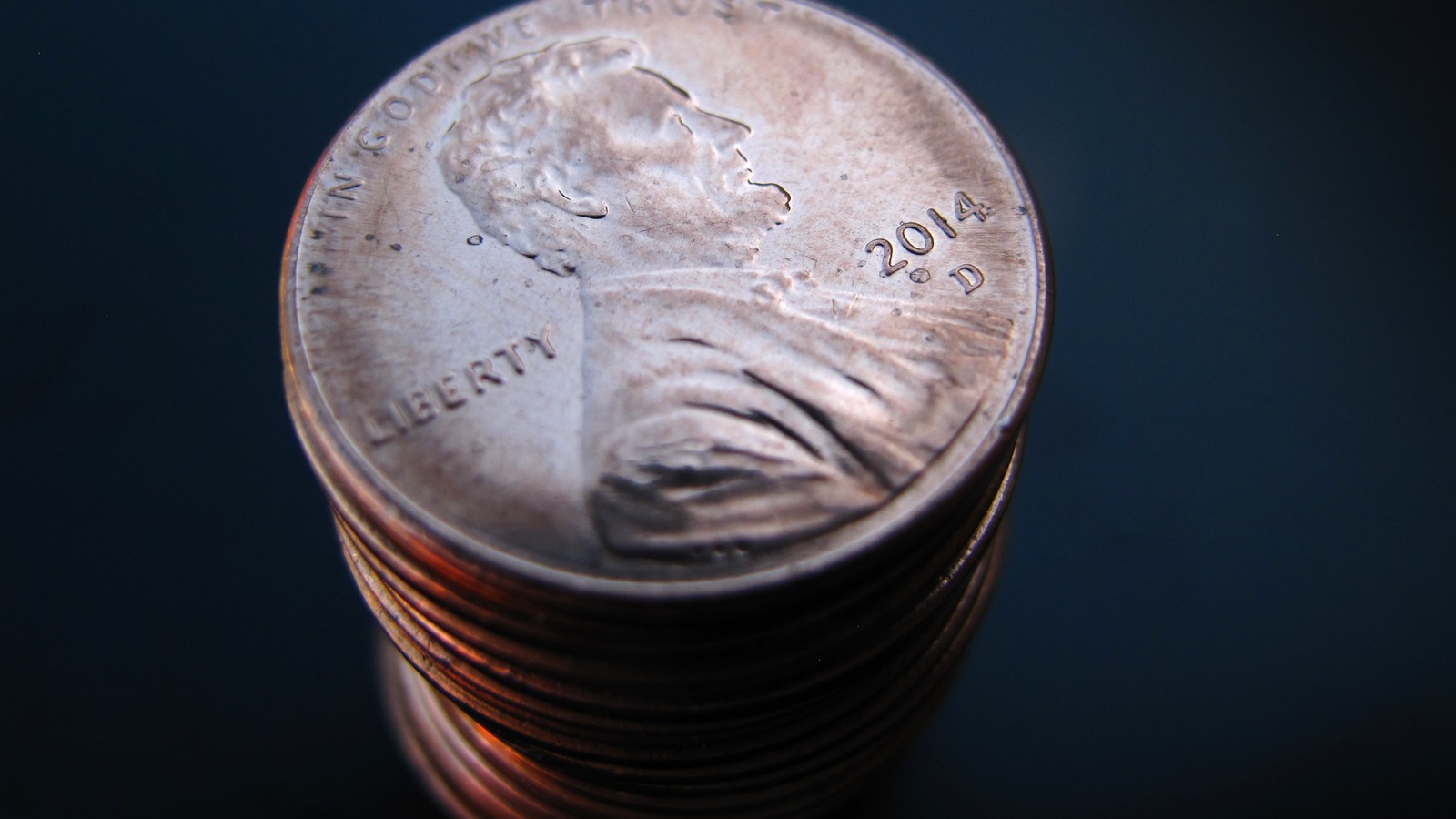This close-up photograph showcases a tall stack of approximately 20 polished, reflective US 1 cent pennies against a navy blue background. Focused primarily on the top penny, it features a side view of Abraham Lincoln, with the word "Liberty" engraved over his left shoulder. The inscription "In God We Trust" arches across the top, though partially obscured. The year "2014" followed by the mint mark "D" is clearly visible in a silvery copper hue at the bottom right. The penny exhibits a mix of shiny and slightly tarnished surfaces, adding depth to its appearance. The photo's angle provides a slight view from above, highlighting the stack's height and capturing the subtle details of the penny's design.